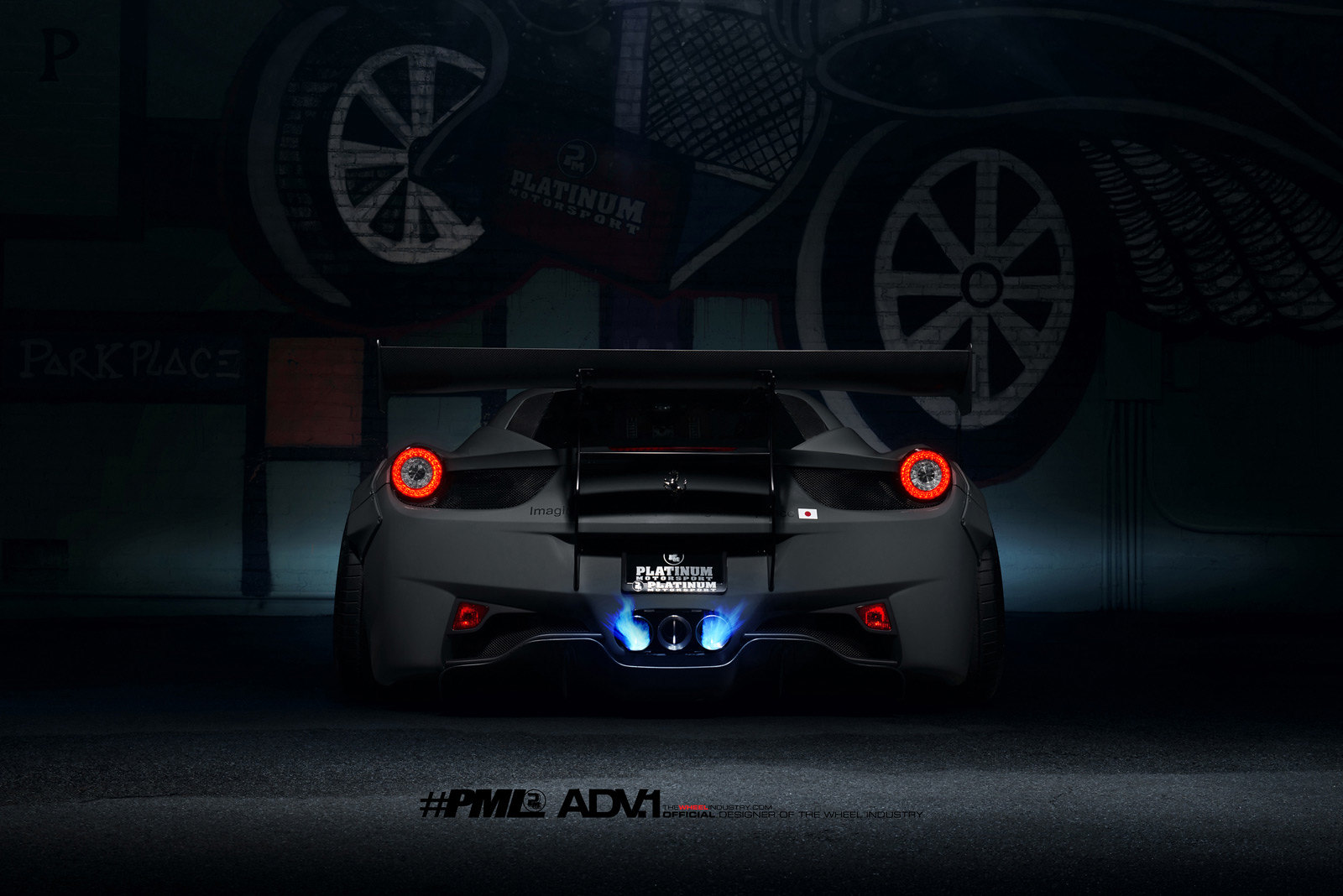In this advertisement, the focus is on the back end of a high-performance gray sportscar. The car is centrally positioned against a dark background, with its two red taillights illuminated and a noticeable silver spoiler on its back. The license plate prominently displays "Platinum" with two bright blue flames shooting from dual exhaust pipes below it. The car’s design is sleek, and it features round red taillights, each encircling unlit white lights. A small Japanese flag is visible on the lower right side of the bumper. The scene depicts the car indoors, perhaps at a car show, with a dark-lit mural as a backdrop, featuring a complex pattern of dark green, orange, and purple squares outlined in black, alongside two painted tires and a banner reading "Platinum Motorsport." Additionally, text at the bottom of the image includes "#PMBADV1," adding to the advertisement’s branding.